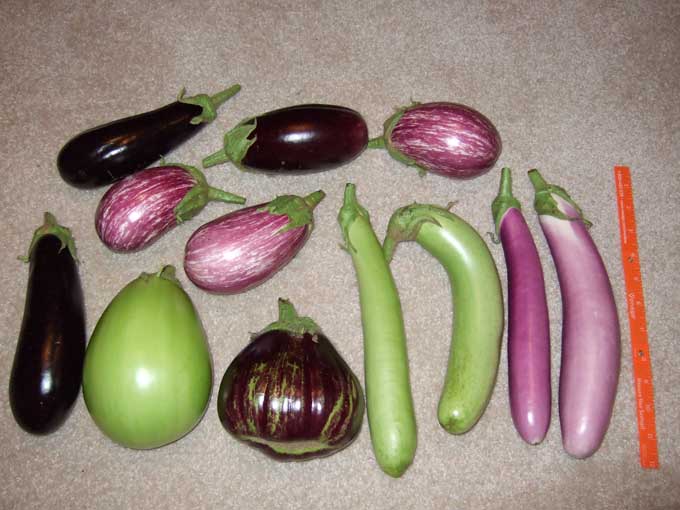The image captures a diverse assortment of 13 eggplants, each exhibiting a range of colors and shapes, splayed out across a beige carpet, reminiscent of one you'd find in an older home. On the right-hand side, a small, thin orange ruler lies adjacent to the eggplants, providing a scale reference. The eggplants vary immensely: there are two with the classic deep purple hue, one slightly paler than the other. There are three longer, green eggplants positioned beside them. Additionally, there is a squat, dark brownish-purple eggplant and another that is green but also flattened. Among the mix are three dark brown, elongated eggplants, and three short, squat ones that are a blend of purplish-white with green stems. The photo suggests these eggplants might represent different varieties or genetic variations, adding to the visual complexity and richness of the scene.